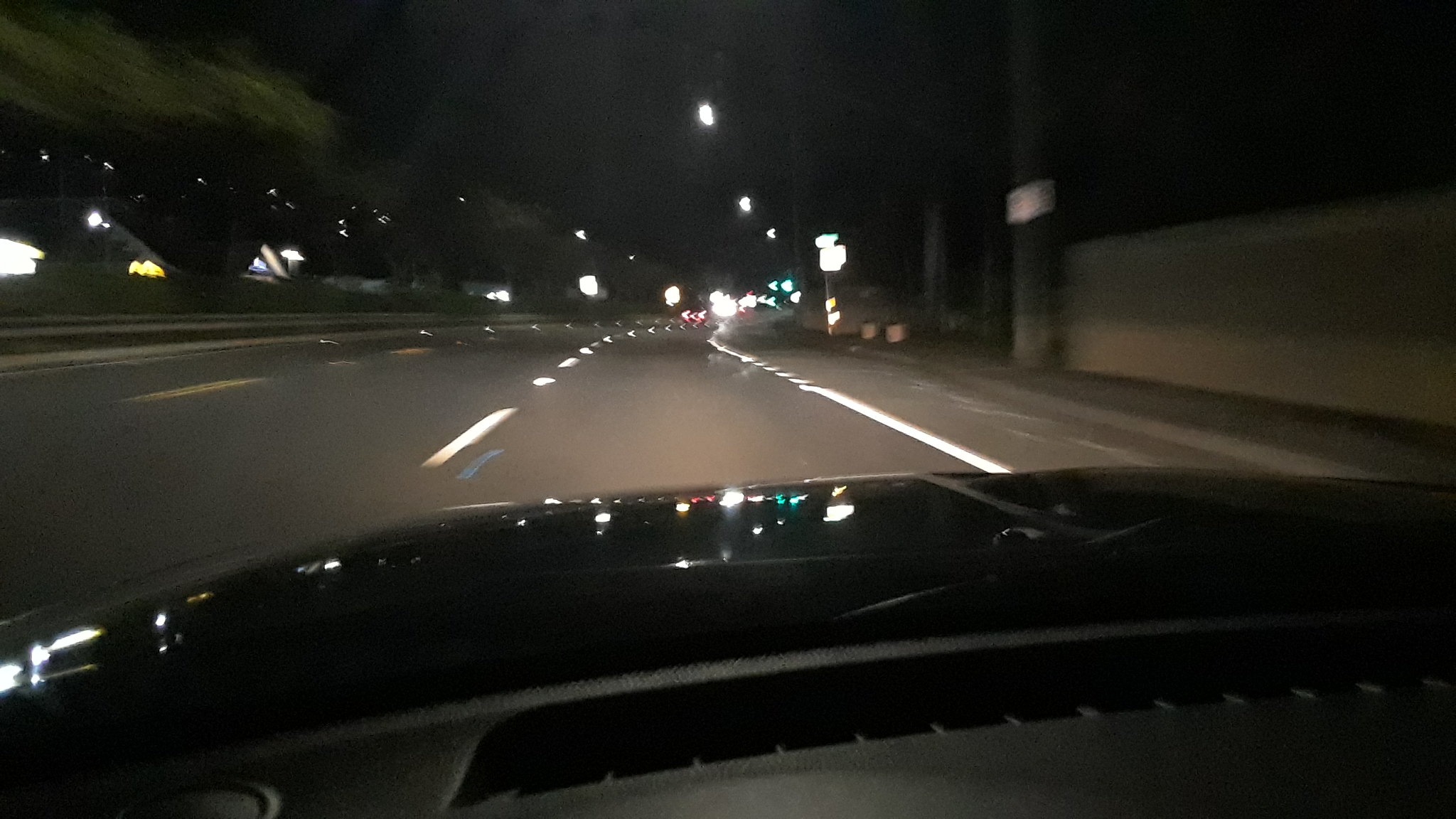A nighttime photograph captured from inside a moving vehicle on a four-lane highway. The scene is illuminated by street lamps lining the road, casting a warm yellow glow. Their light reflects off the hood of the car, which seems to be either black or dark blue. Despite the blur indicating motion, one can clearly see the white lane markings on the asphalt, guiding the way. The overall color palette of the image consists of shades of white, black, gray, yellow, and hints of green, creating a vivid yet moody portrayal of nighttime travel.